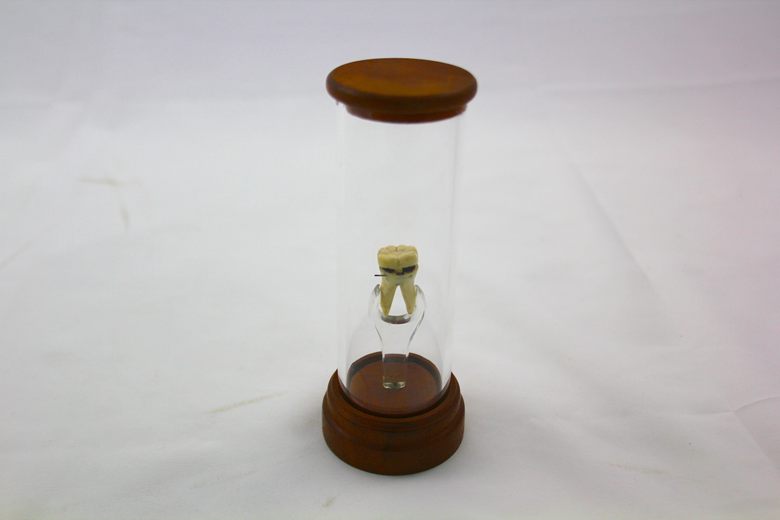This rectangular photograph, wider than it is tall, features a detailed display of a large human tooth encased in a glass container. The background transitions from a grayish hue to a subtle pink on the right side, and the entire scene is set against a white cloth surface that might be a tablecloth or bed sheet. Central to the image is a tall cylindrical glass tube with a dark brown wooden base and matching top. Within this glass enclosure, a clear glass arm, resembling half of a wrench, supports the tooth, which is a beige or whitish-yellow color with distinct dark portions near its middle. The tooth is pointy at both ends and has a horizontal dark line running through it. The overall aesthetic of the display is that of a meticulously crafted exhibit, emphasizing the tooth's detailed structure and coloration.